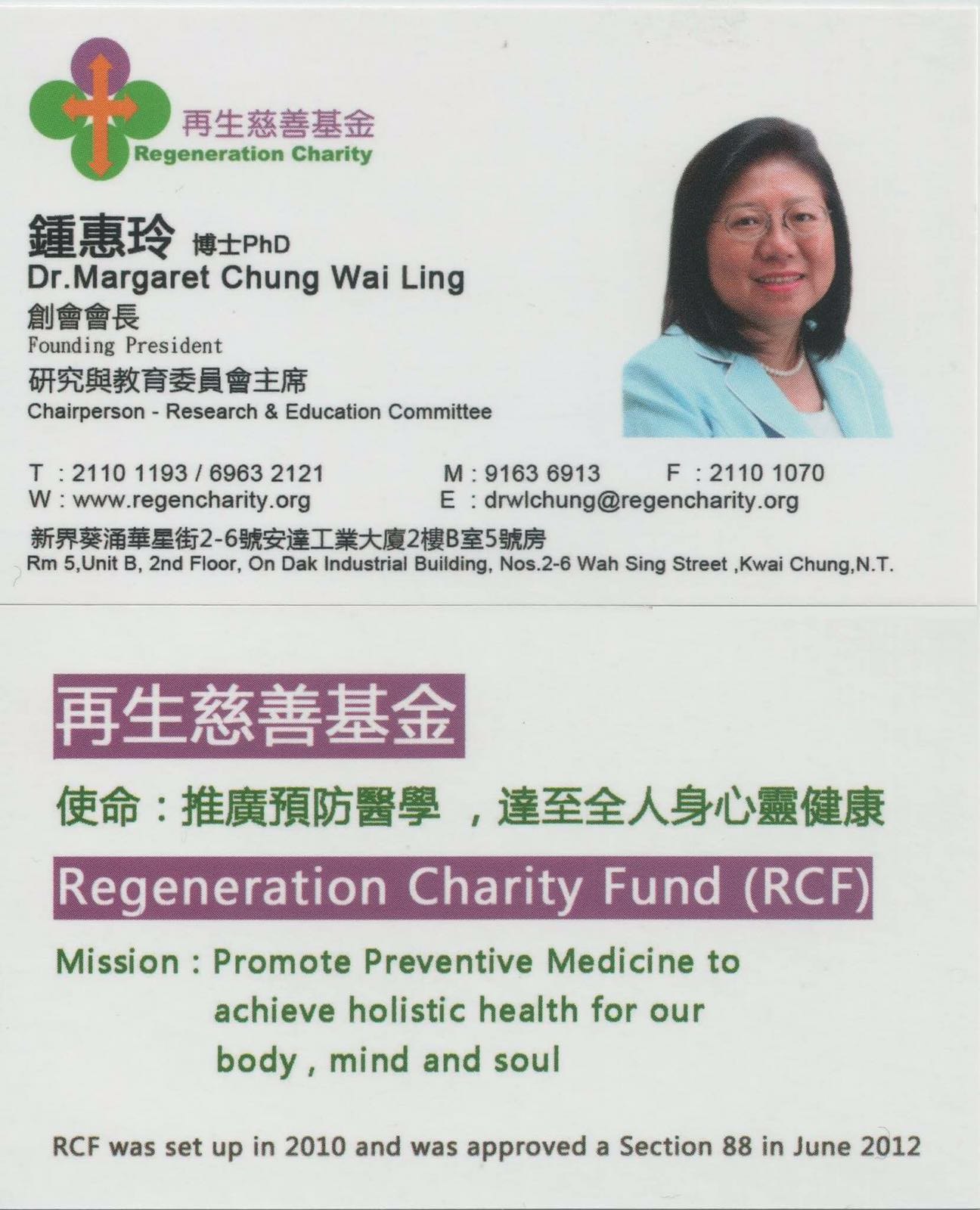The image showcases a detailed business card for Dr. Margaret Chung Wai Ling, founder and chairperson of the Regeneration Charity Fund. The card is divided into two sections: the front and the back. The front presents Dr. Ling's profile, including her credentials as the Founding President and Chairperson of the Research and Education Committee. She is depicted in a profile photo wearing a blue suit jacket, with black, medium-length hair and glasses. Her contact information, including telephone number, website, email, and address (Room 4, Unit B, 2nd Floor, On Deck Industrial Building), are neatly listed. 

The top left corner of the card features the Regeneration Charity logo, which consists of a cross inside four circles—one purple and three green. There is a significant amount of Chinese text, but English is also prominently used throughout. 

On the back, the card outlines the mission of the Regeneration Charity Fund in red text: "Promote Preventative Medicine to Achieve Holistic Health for Our Body, Mind, and Soul." The text explains that the charity was established in 2010 and received Section 88 approval in June 2012. Additionally, the logo incorporating four dots—three green/orange and one blue—centered with uniting arrows is present. This card emphasizes the charity's commitment to preventive medicine and holistic health.